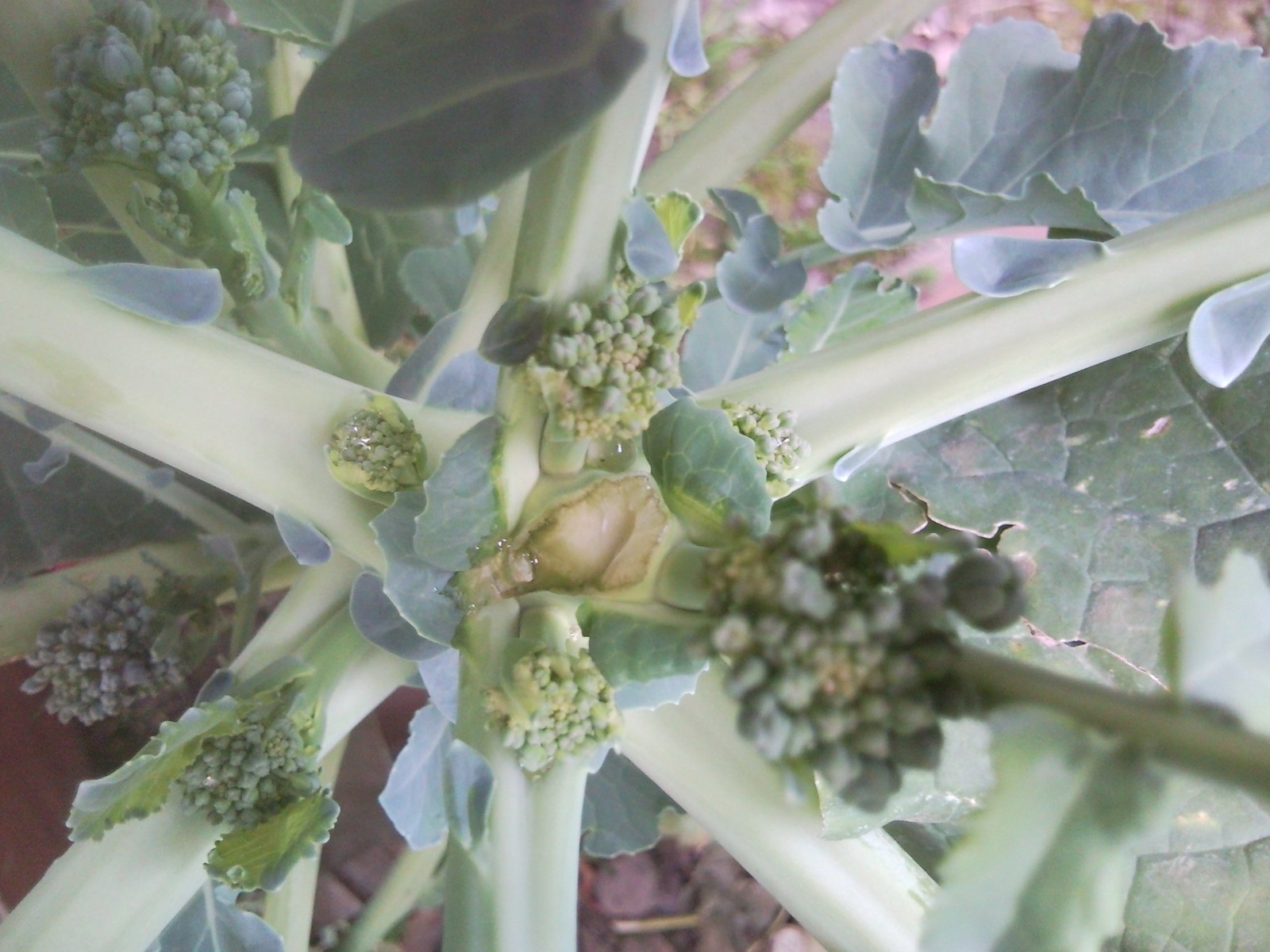This photograph captures a close-up view of a plant that is highly reminiscent of immature broccoli. The picture prominently showcases the thick, pale green stalks that branch out in a star-like pattern, supporting clusters of developing buds. The buds themselves are small, dark green, and beginning to form the familiar rounded shape of mature broccoli heads, interspersed with hints of blue-green and pale yellow. The backdrop comprises numerous green leaves, some of which display brown flecks and signs of insect nibbling, indicative of the plant's growing environment. The overall composition features a somewhat muted and desaturated tone, likely due to the bright but overcast lighting conditions, imparting a grayish cast to the image. The photograph appears slightly blurry and provides a detailed view focused on the central plant, with its thick stems and budding clusters standing out against the backdrop of green foliage.